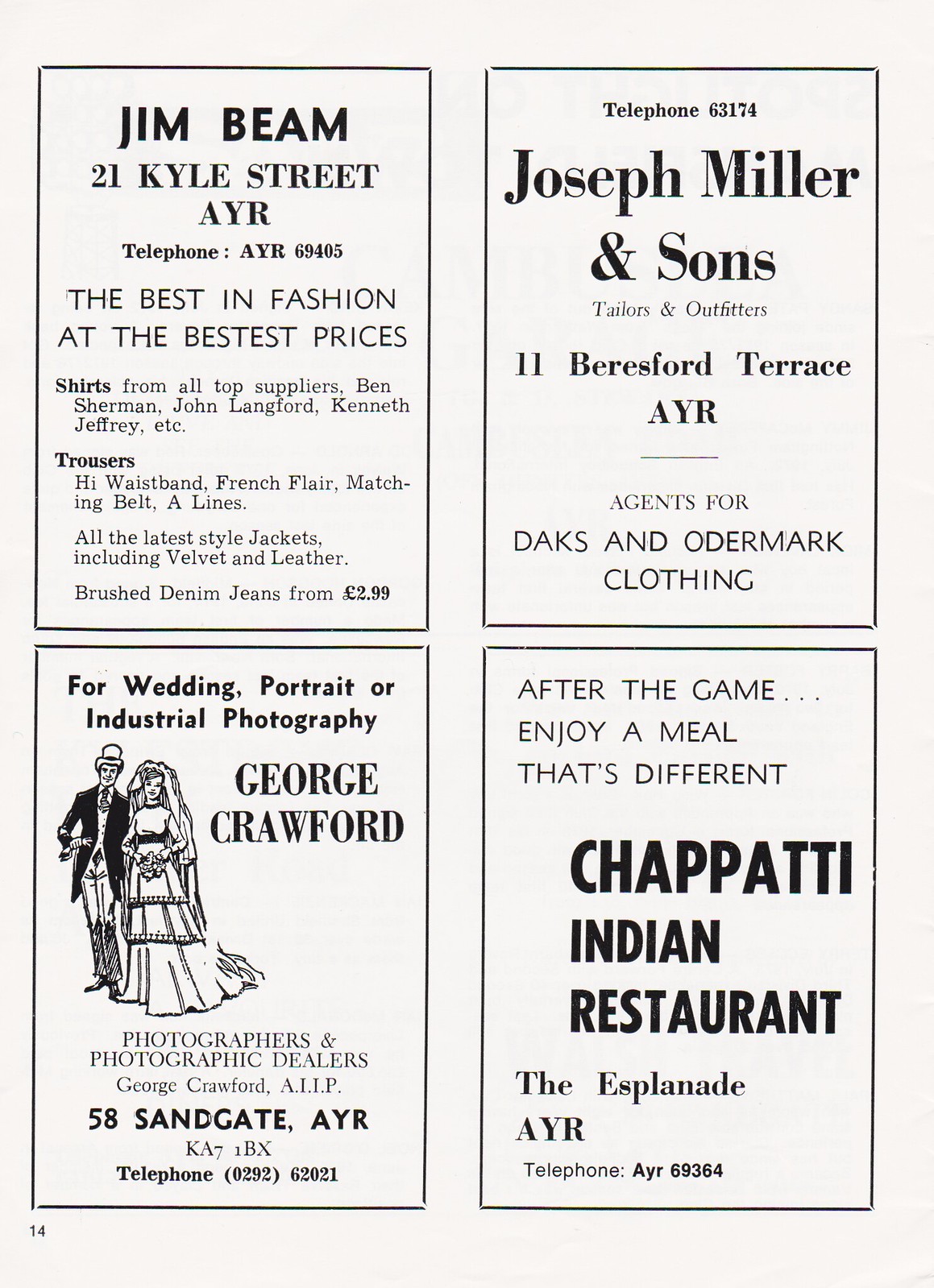This image is an old magazine page divided into four quarters, each containing a detailed advertisement in black lettering on a light blue background. In the upper left corner, the ad promotes Jim Beam at 21 Kyle Street, AYR, and mentions their phone number as AYR 69405. The ad boasts "The best in fashion at the bestest prices," featuring shirts from top suppliers like Ben Sherman, John Langford, and Kenneth Jeffrey. It also highlights trousers with high-waist French flair and matching belts, as well as jackets in the latest styles, including velvet and leather, with brushed denim jeans starting at $2.99.

The top right corner features an ad for Joseph Miller and Sons, located at 11 Beresford Terrace, AYR, with a contact number of 63174. This tailor and outfitter establishment is noted as agents for Dax and Odermark clothing.

On the bottom left, George Crawford’s advertisement offers wedding, portrait, and industrial photography services. It includes a drawing of a bride and groom and provides the business address as 58 Sandgate, AYR, KA7 1BX, with a contact number of 0292 62021. The ad lists George Crawford as an AIIP member and indicates that they are photographers and photographic dealers.

Finally, the bottom right corner promotes the Chapati Indian Restaurant, inviting patrons to "enjoy a meal that's different" after the game. Located on the Esplanade, AYR, they can be reached at AYR 69364.